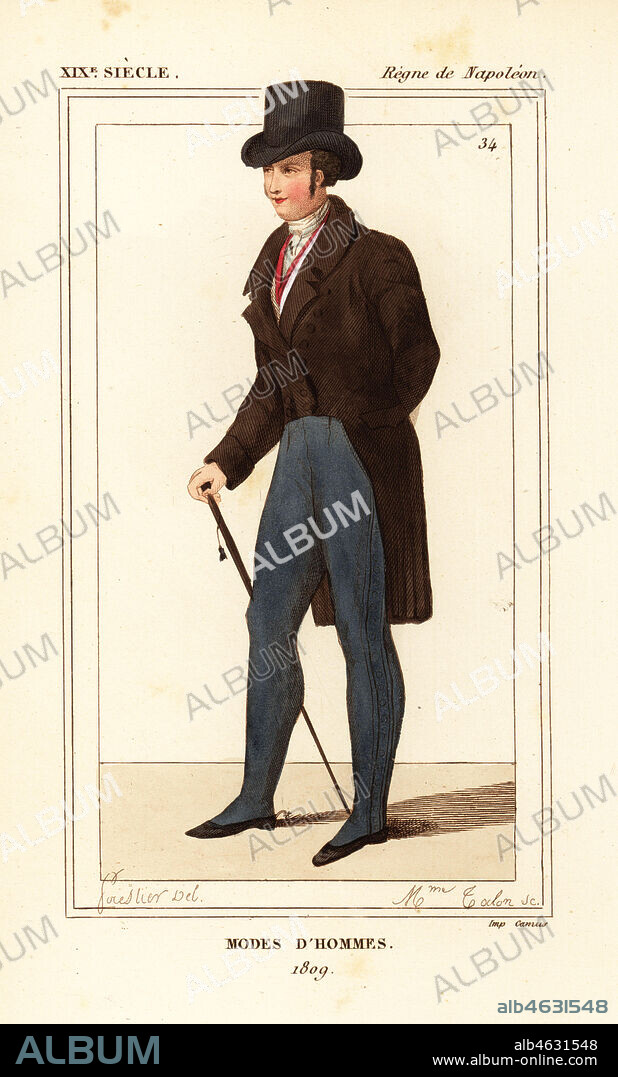This image depicts a man from the early 19th century, adorned in elaborate attire characteristic of the period. He wears a black top hat and a long brown coat, paired with gray pants and slipper-like shoes. A striking red tie or necklace adds a touch of color to his outfit. The man, who has long sideburns and carries a walking stick, exudes an air of elegance and sophistication.

The artwork appears to be a scanned print, featuring various inscriptions. At the top, in cursive writing, the text includes "XIXe Siècle" and "Règne de Napoléon." Below the image, inscribed on a black band, is the title "Modes d'Hommes," dating it to 1809. Additionally, there is a watermark along the bottom of the image, which includes the website "www.album-online.com" and a serial number "A-L-B-4-6-3-1-5-4-8," indicating the image's protected status and available for digital use under certain conditions.